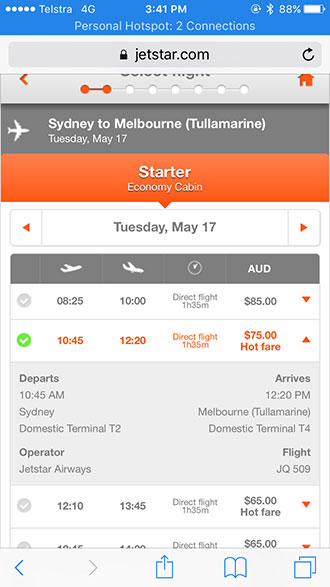This is a detailed screenshot of the Jetstar website, showcasing flight options for a journey from Sydney to Melbourne. Captured on a cell phone connected to a Telstra 4G personal hotspot at 3:41 PM with an 88% battery charge, the image reveals a user browsing Jetstar.com.

At the top of the screenshot, a grey banner plainly states the travel route: "Sydney to Melbourne, Tuesday, May 17th." Just below, an orange banner highlights the cabin class as "Starter Economy Cabin."

The main section provides details on available flights for the selected date:

1. **Flight at 8:25 AM**:
   - **Duration:** 1 hour 35 minutes
   - **Price:** $85
   - **Status:** Not selected

2. **Flight at 10:45 AM** (Highlighted in green as the selected flight):
   - **Duration:** 1 hour 35 minutes
   - **Price:** $75 (labeled as "Hot Fare")
   - **Flight Details:** 
     - **Departure:** 10:45 AM from Sydney Domestic Terminal T2
     - **Arrival:** 12:20 PM at Melbourne Domestic Terminal T4
     - **Operator:** Jetstar Airways
     - **Flight Number:** JQ509

3. **Flight at 12:10 PM**:
   - **Duration:** 1 hour 35 minutes
   - **Price:** Not specified
   - **Status:** Not selected

This thorough screenshot provides comprehensive information on the flight options, assisting users in making an informed decision for their travel plans from Sydney to Melbourne.